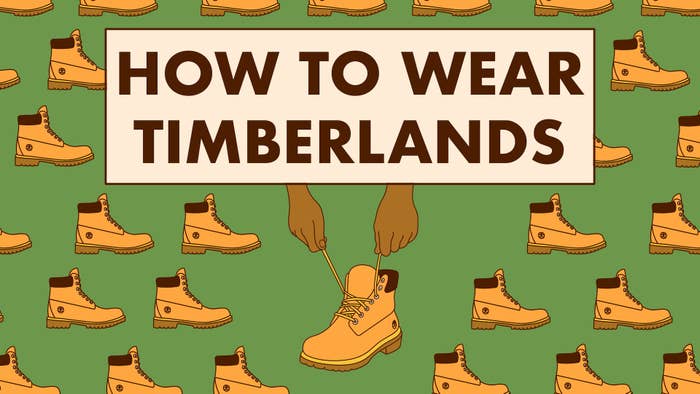This digital illustration portrays a cartoon-style guide on how to wear Timberland boots. The background, a vivid green, is adorned with a repeated pattern of tan-colored Timberland boots, each featuring nubuck leather and a brown leather cup at the top heel area. Every boot showcases a gum-colored sole with a rugged texture. Prominently displayed in the center is a large white rectangular text box with a brown trim. Inside this box, bold uppercase brown letters read "How to Wear Timberlands." Below this text, two black hands are seen holding the laces of a Timberland boot, demonstrating a specific lacing style. The boots, made of yellowish-tan leather, are complemented by their thick, durable soles and ankle-covering design, emphasizing both their iconic style and practical use.